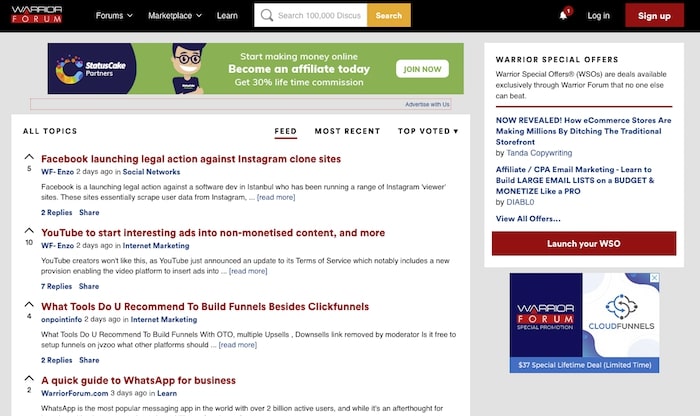The image is a detailed screenshot of a webpage from the Warrior Forum website displayed on a computer screen. At the top of the page, the banner features a black background with the Warrior Forum logo situated in the upper left corner. To the right of the logo, there are several navigation options including a "Forums" drop-down menu, a "Marketplace" drop-down menu, a "Learn" link, and a search bar emblazoned with "Search 100,000 Discussions." The banner also features "Login" and "Sign Up" buttons.

Directly beneath this top banner is another smaller banner which highlights "Status Color Partners" and prominently displays an image of a man sporting eyeglasses, a friendly smile, a dark-colored T-shirt, and black hair, with his arms confidently folded. Accompanying the image is enticing text that reads, "Start making money online. Become an affiliate today. Get 30% lifetime commission." There is also a conspicuous red "Join Now" button.

Further down, the page is categorized by various discussion topics. A navigation menu allows users to filter topics by "Feed," "Most Recent," and "Top Voted." Four selected topics are displayed with brief descriptions:

1. **Facebook launching legal action against Instagram clone sites:** Written in red lettering, posted by WF Enzo two days ago in the "Social Networks" category. The brief excerpt explains Facebook's legal action against an Istanbul-based software developer who operates Instagram viewer sites that scrape user data from Instagram. The post includes options to "Read more," see two replies, and share the discussion.

2. **YouTube to start introducing ads into non-monetized content and more:** Another post by WF Enzo, also from two days ago, this time in the "Internet Marketing" category. It mentions an update to YouTube's Terms of Service that allows the platform to insert ads into videos even if the content isn’t monetized. Users can "Read more," see seven replies, and share the post.

3. **What tools do you recommend to build funnels besides ClickFunnels?:** Posted by On Point Info two days ago in the "Internet Marketing" category. The description suggests a discussion on alternate tools for building sales funnels that include multiple upsells and downsells, although it’s noted the link was removed by the moderator. Users can "Read more," see two replies, and share the post.

4. **A quick guide to WhatsApp for business:** Posted by warriorform.com three days ago in the "Learn" category. The description begins by stating that WhatsApp is the most popular messaging app with over 2 billion users, but it’s cut off after the first line. Options to "Read more," see replies, and share are also present.

On the far right, there is a column dedicated to "Warrior Special Offers" (WSOs). This section explains that WSOs are exclusive deals available only to Warrior Forum members. Featured offers include:

1. **How e-commerce stores are making millions by ditching the traditional storefront:** by Tanda Copywriting.
2. **Affiliate/CPA email marketing:** Learn to build large email lists on a budget and monetize like a pro by Diablo.

Additionally, there are options to "View all offers" or "Launch your WSO."

At the very bottom of the screenshot, the logos for Warrior Forum and Cloud Funnels are displayed along with a promotional offer: a $37 special lifetime deal available for a limited time.